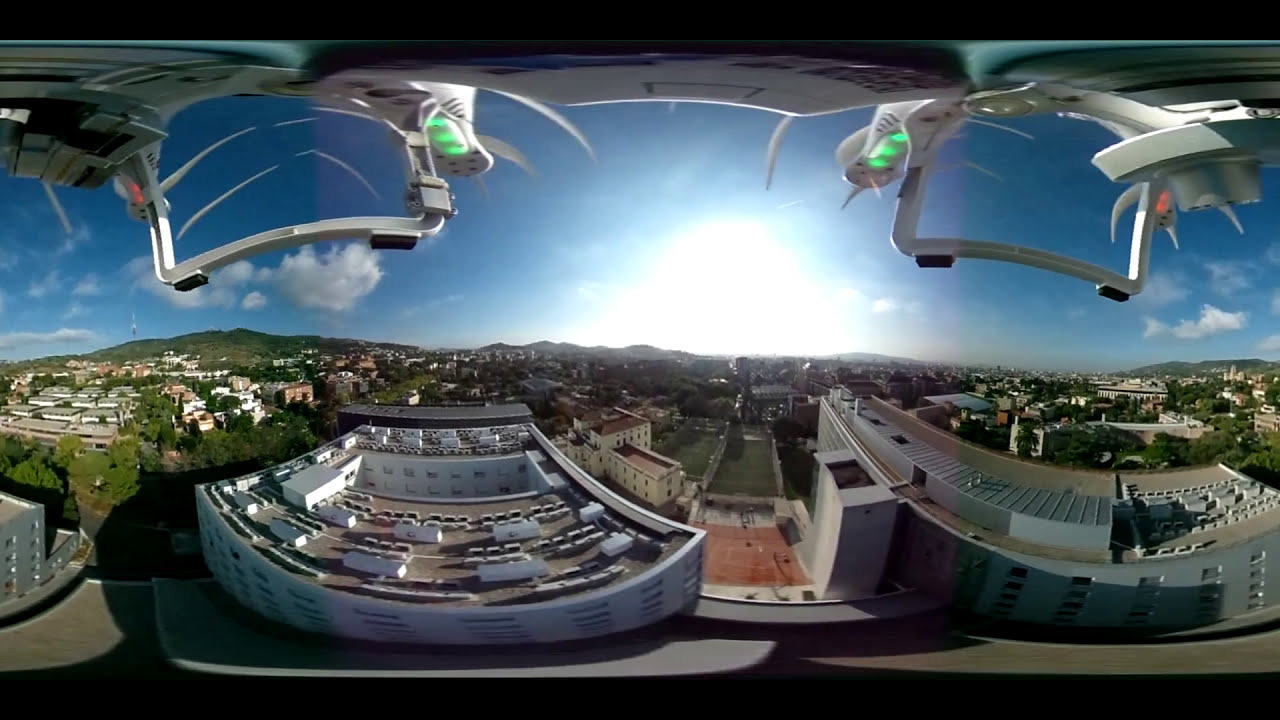The image is an impressive 360-degree aerial panorama captured by a drone, showcasing a blend of urban and natural landscapes. At the top of the image, there is a thin black border framing the view. The drone, a white model with green and red lights, is visibly positioned at the image's top edge, with its propellers and landing struts partially in view.

In the background, half of the image reveals a blue sky dotted with white clouds and dominated by a brilliantly shining sun at its center, casting bright white glare. Below the drone, a sprawling cityscape unfolds. In the center, there is a prominent square apartment building surrounded by various multi-story structures with flat roofs. Here, you can spot a football field and a basketball court adorned in orange. The city is interspersed with abundant greenery, featuring numerous trees.

On the horizon, extending across the background, are hills or mountains that add a picturesque touch to the setting. The sunlight creates noticeable shadows, indicating the photo was taken in the bright light of midday. The colors in the image range from the natural greens of the trees, various shades of blue in the sky, and the tans and whites of the buildings, to the vivid lime green and orange of certain features.

Overall, this detailed aerial view captures a harmonious blend of urban and natural elements under a bright, midday sky, framed by the body's drone structure.